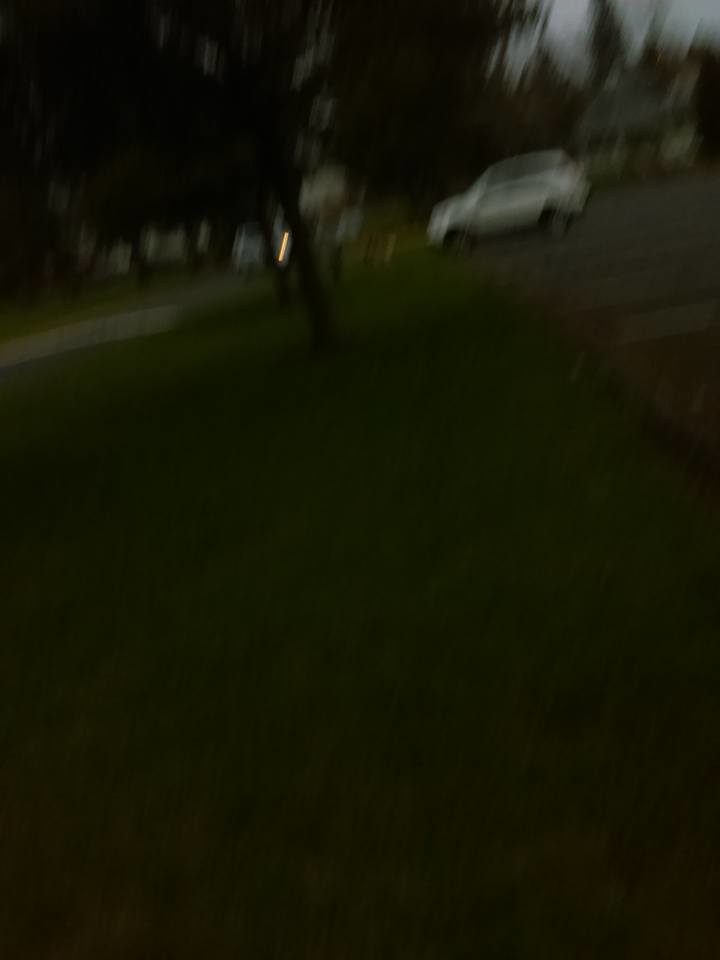A blurry image depicts a scene with indistinct elements. In the background, trees with leafy canopies are faintly visible. A van is the primary focus, with its form partially discernible amidst the blurriness. To the right, there's a suggestion of a road or possibly a parking lot, characterized by a mix of asphalt and grass. Additional vehicles can be seen in the distant, obscure background, adding to the scene's overall sense of motion and activity. Despite the indistinct quality, the image evokes a bustling yet serene roadside or park setting.